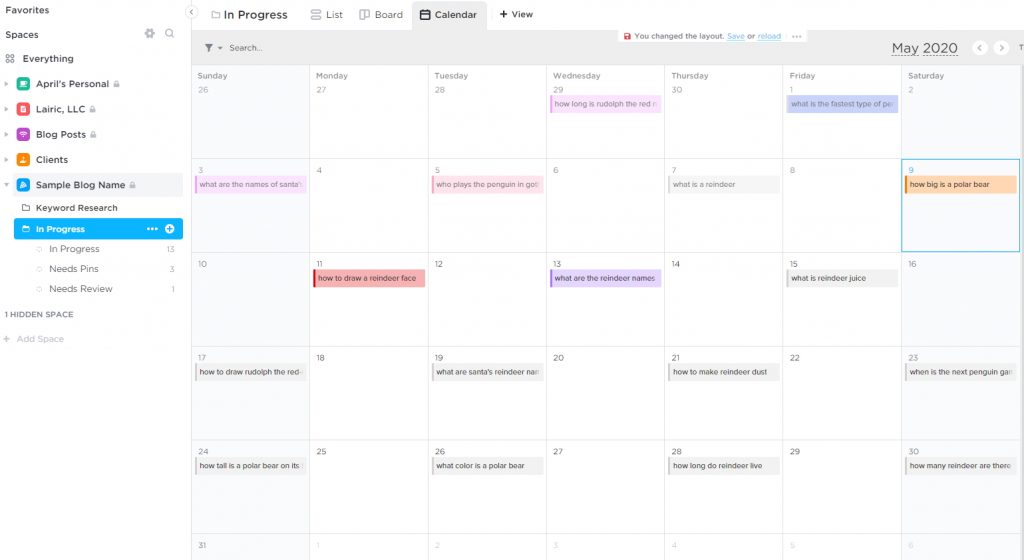This image is a detailed screenshot from a computer or laptop with a landscape orientation, set against a predominantly white backdrop interspersed with various colors. On the left-hand side, there is a vertical white toolbar with a black header labeled "Favorites." Beneath this header are several categorized and color-coded sections: "Everything" followed by "April's Personal" in green, "Lyric LLC" in red, "Blog Post" in purple, "Clients" in orange, and "Sample Blog Name" in blue. Below these sections, there is an entry titled "Keyboard Research" in black, and an "In Progress" bar highlighted in blue with white text. The subheaders within this section include "In Progress," "Needs Pins," and "Needs Review."

To the right of the toolbar is a calendar interface with a header that reads "In Progress" and options to view the content in a "List," "Board," or "Calendar" format. The "Calendar" view is currently selected and highlighted in gray. This calendar spans from Sunday, May 26th to Saturday, May 30th. Various events are indicated with color-coded boxes corresponding to the categories listed on the toolbar. Notably, on Saturday, May 9th, there is a prominent event marked with an orange box and black font surrounded by a blue border, indicating an important event.